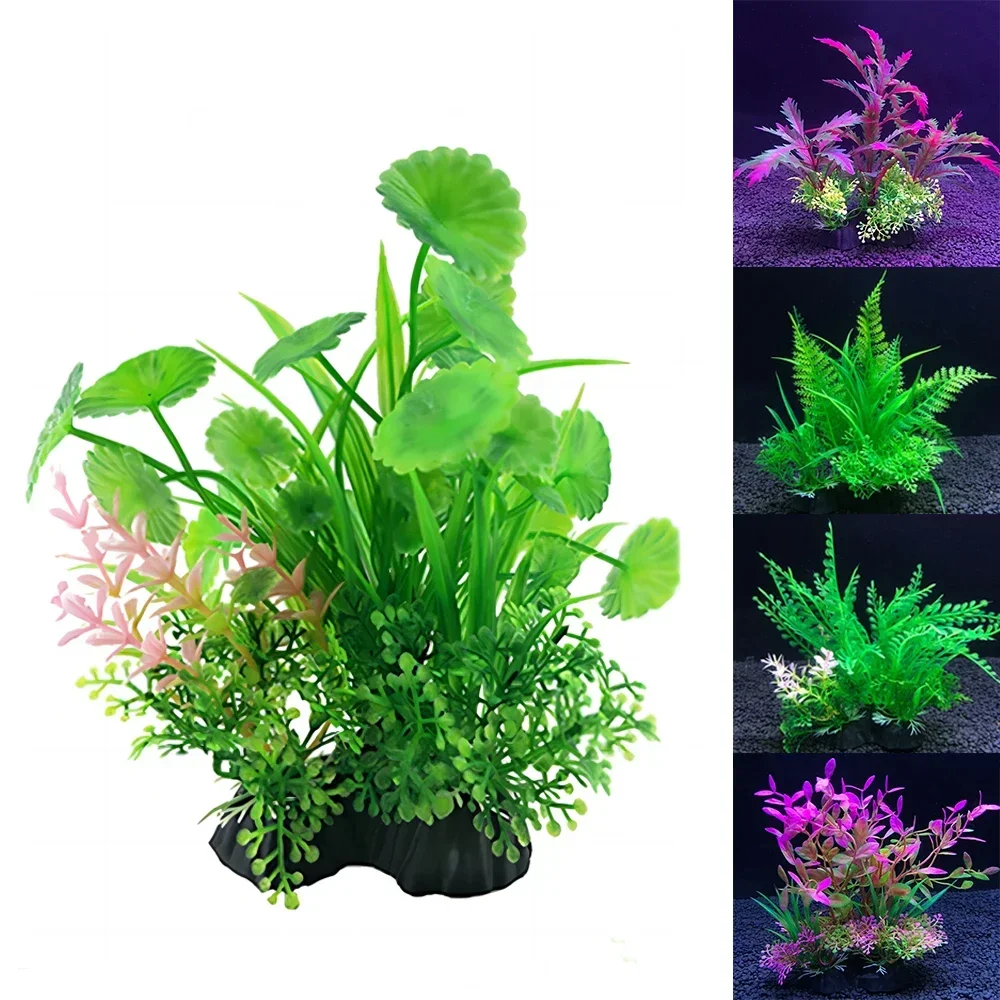The image appears to be a promotional photo for a product, possibly from Wish or Teemu, showcasing a collection of artificial aquarium plants. The main attraction on the left side of the image is a single large plasticky green plant adorned with several pink blossoms. This plant is placed above a small plastic rock or a black C-shaped stump. Surrounding it are several grass-like shoots. 

On the right side, there are four smaller images of additional plants arranged in a vertical sequence:

1. The top image features a reddish-purple plant with light green leaves, set against a purple backdrop and ground, possibly due to overhead lighting. Small white flowers are interspersed among the leaves.
2. The second image displays a green plant with firm, kelp-like leaves set against a black background and black floor.
3. The third image shows another green plant, similar to a fern, positioned against a black background and gray rocks. This plant is accented by small white flowers emerging from the left side.
4. The fourth and bottom image consists of a purple plant with green leaves, arranged against a black background with dark blue rocks.

All the plants showcased in this image have a notably artificial appearance, resembling common decorations used in aquariums for aesthetic enhancement and to provide an environment for fish to swim around. There are no texts or labels in the picture, emphasizing the visual representation of the products.